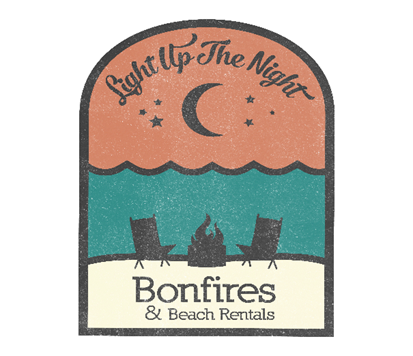This image depicts a detailed logo or business sign shaped like a doorway with an arched top, transitioning to a straight bottom. The top third of the sign features an orangey, faded red background and prominently displays the phrase "Light Up The Night" in black, cursive lettering that follows the curve of the arch. Centrally positioned within this top section is a black crescent moon, flanked by three stars on each side, arranged in a triangular pattern.

Below this, a blue-green band represents water, with wave-like detailing at its upper edge. In the middle of this section, two blacked-out beach chairs are facing each other, centered around a black bonfire.

The bottom third of the logo is bordered by a sandy or whitish-yellow background. This section features the text "Bonfires and Beach Rentals," with "Bonfires" written more prominently in black. The entire design is outlined in a thin black border, ensuring all elements are center-justified and harmoniously blended within the logo.